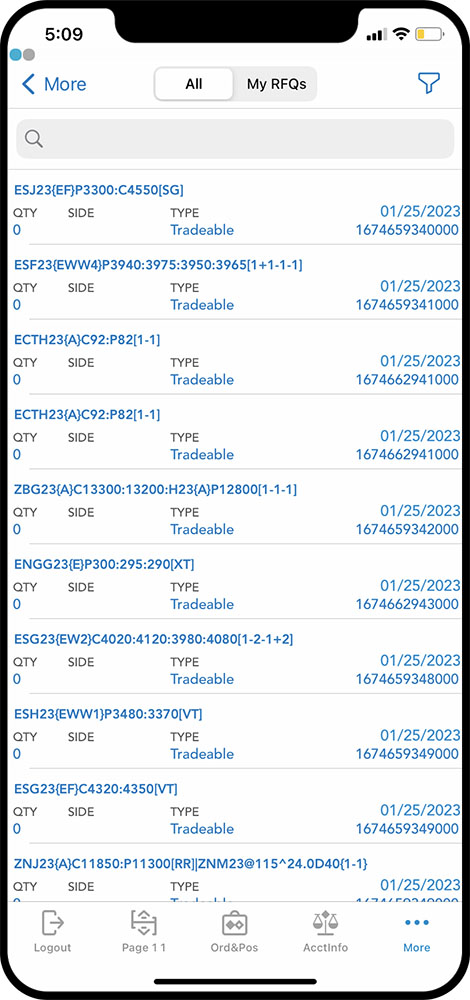This is a screenshot of a mobile phone displaying a table with four columns, showcasing text in blue and grey. At the top of the screen, there's a 'back' arrow and the word 'More' in blue. The center displays a tab currently switched on, labeled 'My RFQs', and on the extreme right is a filter icon. Below this, there is a grey search bar. Underneath the search bar, the table itself is displayed. Each row in the table begins with a long serial number, followed by four columns. The column headers in black font read: 'Quantity', 'Price', 'Type', and 'Date'. Each row repeats a serial number beneath these headers. At the bottom of the screen are five icons: a 'Logout' icon, a 'Page' icon, an 'Award and Post' icon, an 'Act Info' icon, and three dots accompanied by the word 'More'.